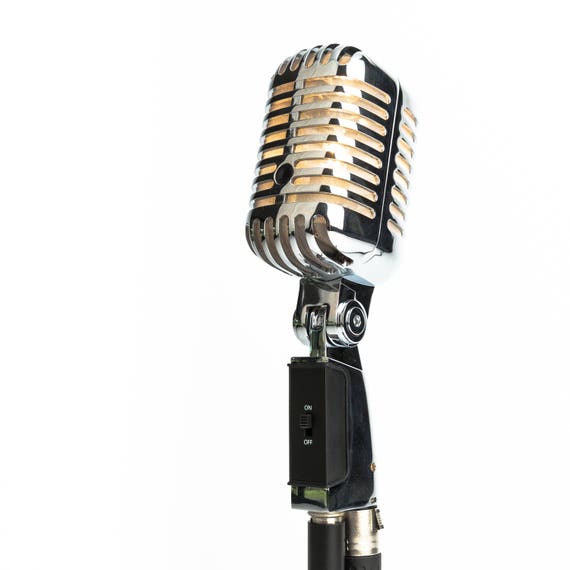This color photograph features a vintage-style cardioid microphone positioned on a black and silver mic stand against a plain white background. The microphone itself boasts a shiny chrome body with distinctive rectangular slits arranged horizontally on its broad, rectangular top. A golden or bone-white color material is visible through these slits, enhancing its retro aesthetic. The microphone's frame is accentuated by black elements, including a black switch panel located on the neck of the stand, marked with 'ON' at the top and 'OFF' at the bottom. A silver and black hinge connects the microphone head to its neck, allowing it to swivel. The setup evokes an era reminiscent of the 1940s, suggesting it could be used for addressing groups of musicians, disc jockeys, or classic crooners.